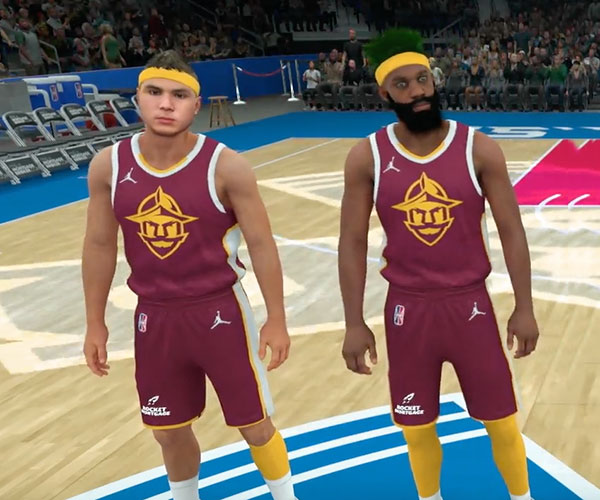This image captures two basketball players standing on a light brown court outlined in blue, with a vibrant crowd of fans in the background. Both players are donning maroon sleeveless jerseys and matching shorts, accessorized with white and yellow socks and yellow headbands. The player on the left, who appears to be Hispanic, has short brown hair, muscular arms, and a serious expression as he stares directly at the camera. The player on the right is African-American, sporting a unique look with hair standing straight up and a rich mossy green color, along with intense, wide-open green eyes that give him a fierce appearance. Their jerseys feature an image of a player stretching out in midair on the top left side of their chests and a gold Viking figure in the center. There is also a white stripe down the side of their shorts, with the word "Rocket" partially visible at the bottom of their right leg.